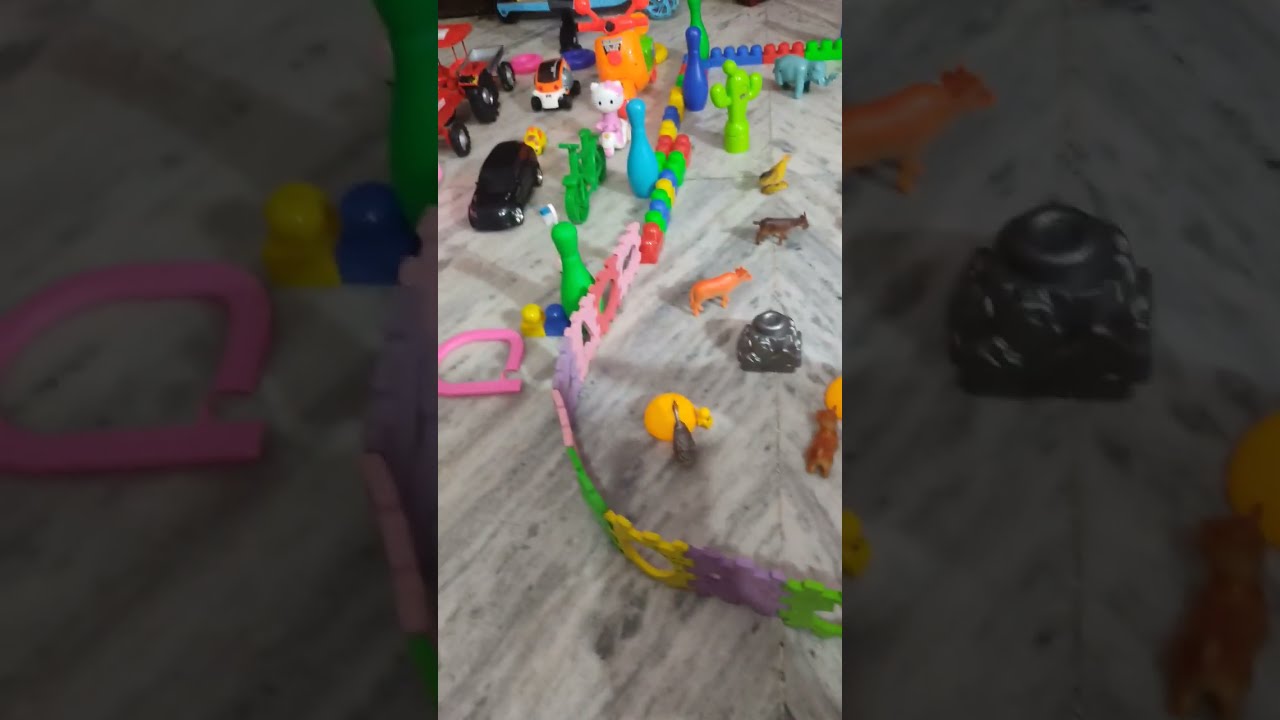The photograph is a horizontal rectangle, structured into three vertical sections. The central vertical section is in clear focus, while the left and right sections are slightly blurred. The scene appears to be a collection of children’s toys meticulously arranged on a gray and white marbled tile surface, possibly a table or floor. The array of colorful toys includes a black car, a red tractor, and a smaller car situated in the upper left corner. Behind these, more toys like a Mr. Potato Head and a white cat figure are visible. A green motorcycle and a green bowling pin are also present, with an assortment of linked colorful pieces akin to a domino effect spread out. Additional bowling pins, including light blue and dark blue ones, can be seen in the background. On the right side, there is a toy cactus and various toy animals. The left and right blurred sections show additional toys and hints of light-colored surfaces. The blurred sections frame the detailed central view, emphasizing the vibrant, playful scene with no visible text or human figures, giving an impression that the setup is indoors, possibly in a home or a school setting.